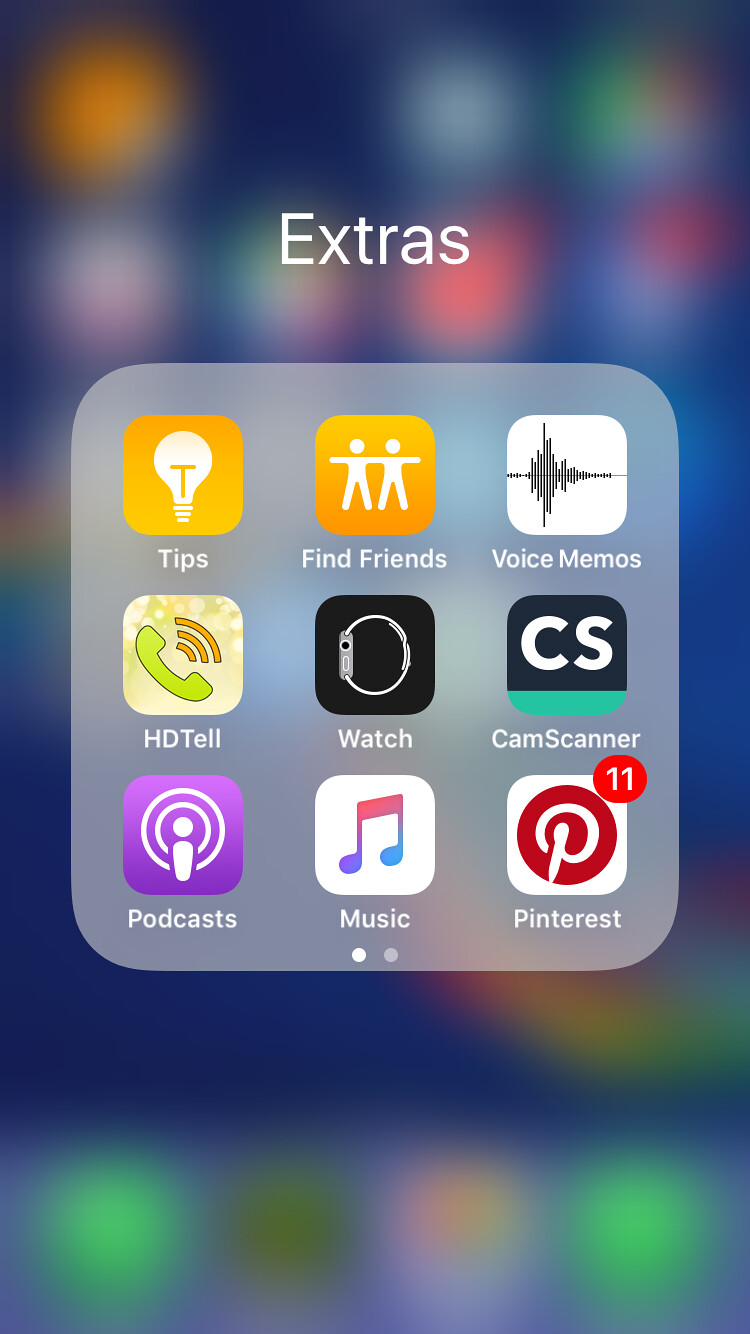The image is a rectangular screenshot of a smartphone interface. The longer sides of the image are the left and right edges, while the shorter sides are the top and bottom edges. The background features a dark blue wallpaper with multiple brightly colored, blurred icons, suggesting it is the desktop of the smartphone.

At the top of the image, there is a clear and focused line of white text that reads "Extras." Dominating the center of the image is a gray, semi-transparent square with rounded corners, presenting a neat grid layout for various applications. This grid consists of three rows and three columns, each icon accompanied by white text labels.

Beginning from the top-left corner of the grid, the first icon is an orange square with a white light bulb, labeled "Tips." Next, to its right, is another orange square featuring the outlines of two people, labeled "Find Friends." Further right is a white square with multiple black lines, labeled "Voice Memos."

In the second row, the leftmost icon is a green square with a green phone icon, labeled "HD Tell." To its right is a black square displaying the side profile of a smartwatch, labeled "Watch." The snapshot ends before completing details for the next icons in the grid, focusing on these mentioned applications.